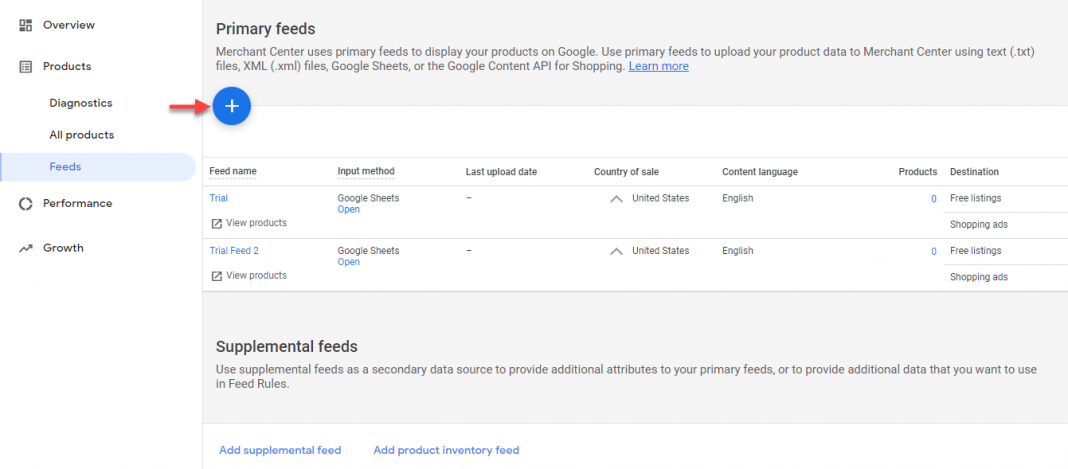**Descriptive Caption:**

The image is a detailed screenshot of the Google Merchant Center’s interface, specifically focusing on the 'Primary Feeds' section. On the left-hand side, there is a navigation menu with the following items: Overview, Products, Inset, Drop-down, Diagnostics, All Products, and Feeds. 'Feeds' is highlighted in blue with a corresponding blue bar to its left.

In the main area, titled 'Primary Feeds', a blue circular button with a plus sign is prominently highlighted by a red arrow added to the image. The text under the 'Primary Feeds' header reads, "Merchant Center uses primary feeds to display your products on Google. Use primary feeds to upload your product data to Merchant Center using .txt files, .xml files, Google Sheets, or the Content API for Shopping." There is a hyperlinked text 'Learn more' highlighted for additional information.

Below the introductory paragraph, there are several columns with headers: Feed Name, Input Method, Last Upload Date, Country of Sale, Content Language, Product and Destination. Two trial feeds are listed: 'trial' and 'trial feed 2', both using Google Sheets as the input method, with 'US' as the country of sale, 'English' as the content language, zero products listed, and destinations being 'Free Listings' and 'Shopping Ads'.

Further down, the 'Supplemental Feeds' section is explained with the text: "Use supplemental feeds as a secondary data source to provide additional attributes to the primary feed or to provide additional data that you want to use on your feeds." Below this, there are links to 'Add Supplemental Feed' and 'Add Product Inventory Feed'.